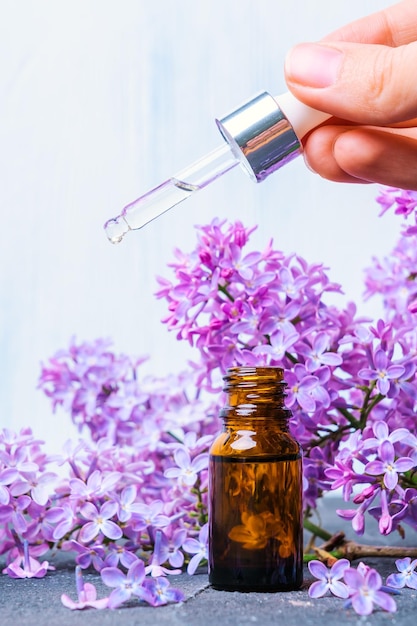This photograph captures a detailed and vibrant scene. An amber bottle, almost completely full of clear liquid, sits on a textured dark gray surface. In the upper right corner, a Caucasian hand holds an eyedropper with a white handle and a thick silver ring. The clear dropper tube is about half-filled with the liquid, and a drop is just beginning to form at its tip. Behind the bottle and dropper, a display of freshly picked purplish-pink and fuchsia flowers, possibly lilacs or forsythia blossoms, creates a beautiful and fragrant backdrop. Some blossoms have fallen onto the surface around the bottle. The background behind these flowers is a pristine white, enhancing the vivid colors of the scene. The bottle, hand, and dropper are in sharp focus, emphasizing their details against the soft, slightly blurred floral background.